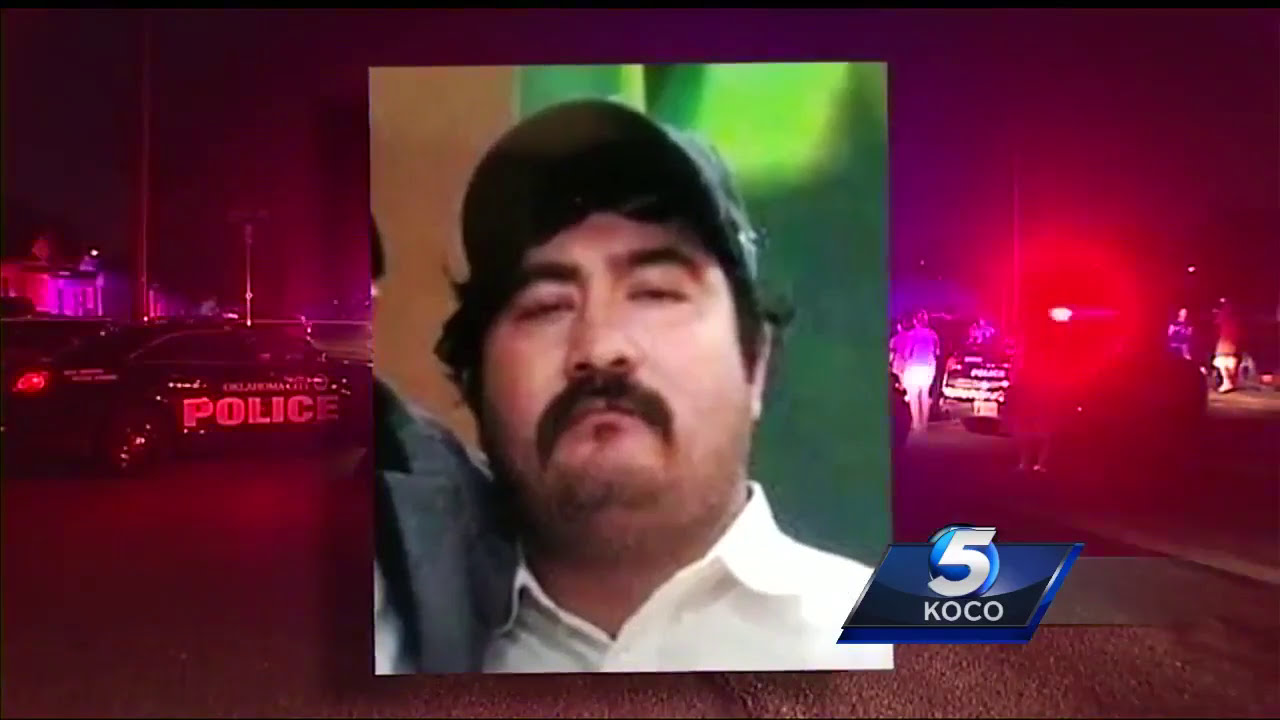The image is a detailed screenshot from a local news broadcast by 5KOCO, depicting a police scene at night. Dominating the center of the image is an inset picture of a Hispanic man with a black mustache, dark hair, and a gray ball cap, wearing a white button-down shirt. The surrounding scene, bathed in a red hue from emergency lights, shows several police cars and a few individuals standing near houses. The KOCO logo, featuring white text with dark and light blue elements, is positioned at the bottom right of the man's picture. The man's eyes are partially closed, and he appears somewhat stout. The background suggests a serious incident or crime, with visible officers and ongoing investigation activities.